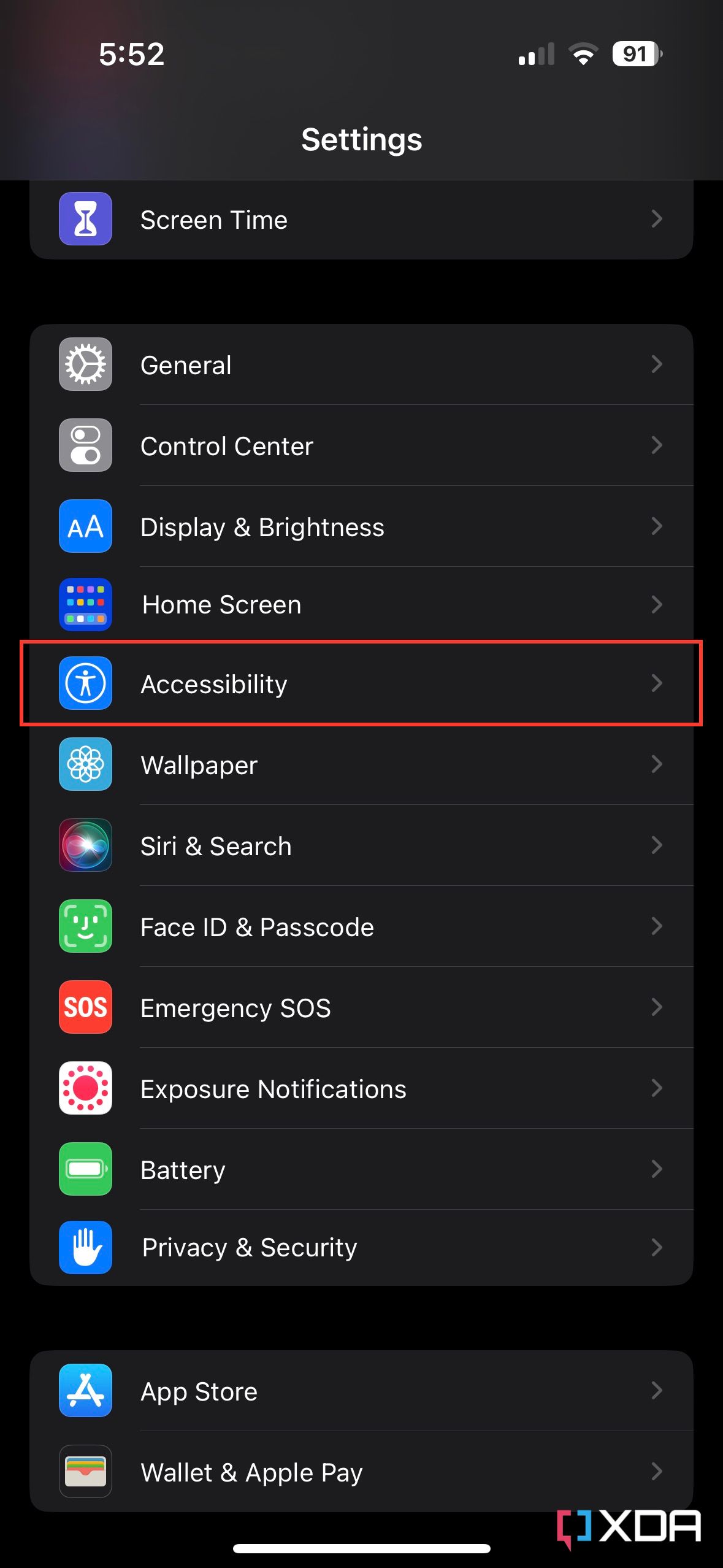The image is a detailed screenshot taken on an iPhone, displaying the iPhone settings menu in dark mode. At the top of the screen, the time is shown as 5:52 on the left, while on the right, icons indicate a connection, WiFi strength, and battery percentage. The visible sections of the settings menu include options such as Screen Time, General, Control Center, Display & Brightness, Home Screen, Accessibility, Wallpaper, Siri & Search, Face ID & Passcode, Emergency SOS, Exposure Notifications, Battery, Privacy & Security, App Store, and Wallet & Apple Pay. The Accessibility option is highlighted with a rectangular box, potentially indicating its importance or focus of the screenshot. The black background confirms that the device is in dark mode. This image might be illustrating how to access or change certain settings on the iPhone, possibly extracted from a video tutorial.